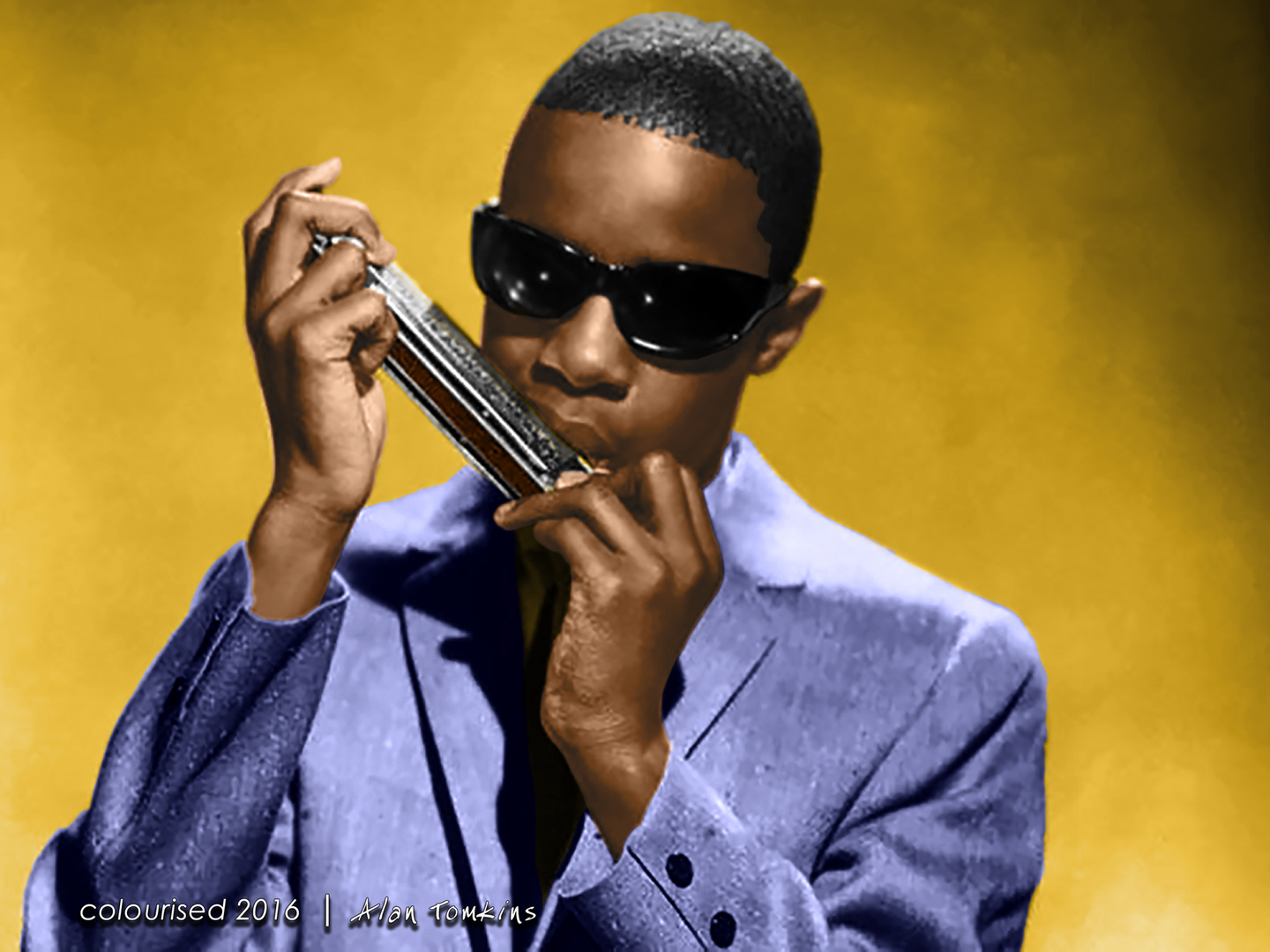In this color photograph, a man with short black hair is captured playing a large silver harmonica. He is wearing sharp black wraparound sunglasses that cover his entire eyes, giving him a striking appearance. His outfit consists of a blue jacket, which appears grayish-blue in some areas, over a black shirt, and possibly a tie. The harmonica, held firmly with both hands, is positioned with the higher end pointing towards the top left of the image as he blows into it. The background is predominantly yellow, with a slight darkening towards the upper right-hand corner. In white script at the lower left-hand corner, the text reads "colorized, 2016," followed by a vertical line and the name "Elon Tompkins."